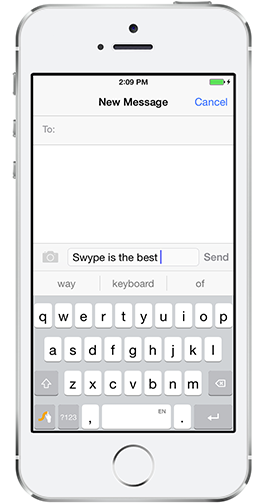The image depicts the front view of an iPhone 8 Plus, encased in a sleek silver border with a white plastic exterior. The phone's screen is active, displaying a rich interface filled with details. At the top left corner of the screen, the time reads from 2 a.m. to 9 p.m., indicating perhaps an active Do Not Disturb schedule or a similar notification setting. The phone shows full bar cellular coverage and indicates a full charge with a green battery icon. 

Prominently displayed in the text messaging interface, a message draft field shows the prompt "Need message" with a blue "Cancel" option beside it. The text field itself is currently blank. There is a nearby camera symbol with the phrase "Swipe is the best" typed just next to it. A "Send" button is located alongside this text field. Below this text field, AI-generated text suggestions read "way," "keyboard," and "of."

The virtual keyboard occupies the lower half of the screen, with all the keys presented in white and the letters in black. There is a gray arrow-up symbol for capitalization, a gray backspace icon, and an unspecified icon featuring an orange "S" located below the backspace key. At the very bottom of the screen, the familiar circular Home button, embedded within the phone's bezel, is visible and ready for fingerprint identification.

This detailed view provides a comprehensive glimpse into the phone’s usage and settings, reflecting a typical text messaging session on an iPhone 8 Plus.